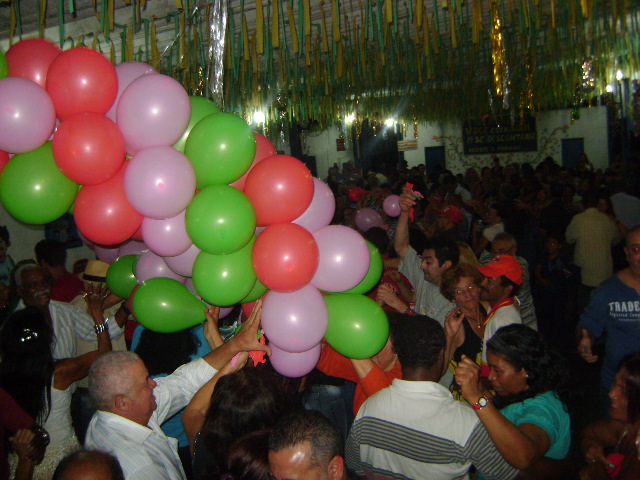The image showcases a lively indoor party scene with several people dancing and celebrating. The ceiling is adorned with festive designs in yellow, green, gold, and silver, which include streamers and banners contributing to the cheerful atmosphere. A cluster of balloons in green, pink, and red hues is prominently displayed in the middle-left portion of the image. Among the attendees, a woman with green-painted nails can be seen smiling at the bottom right of the picture. Nearby, a woman in green, wearing a red watch and dancing with a man, adds to the vibrant activity. In the center, a man is captured with one hand raised, enhancing the dynamic feel of the scene. The background features a wall decorated with a banner, adding to the celebratory decor. The image overall is well-lit, thanks to natural light, contrasting with the dimly lit room. In the foreground, a man wearing a white shirt with black stripes is dancing with a woman in a blue shirt, accentuating the joyous essence of the gathering.